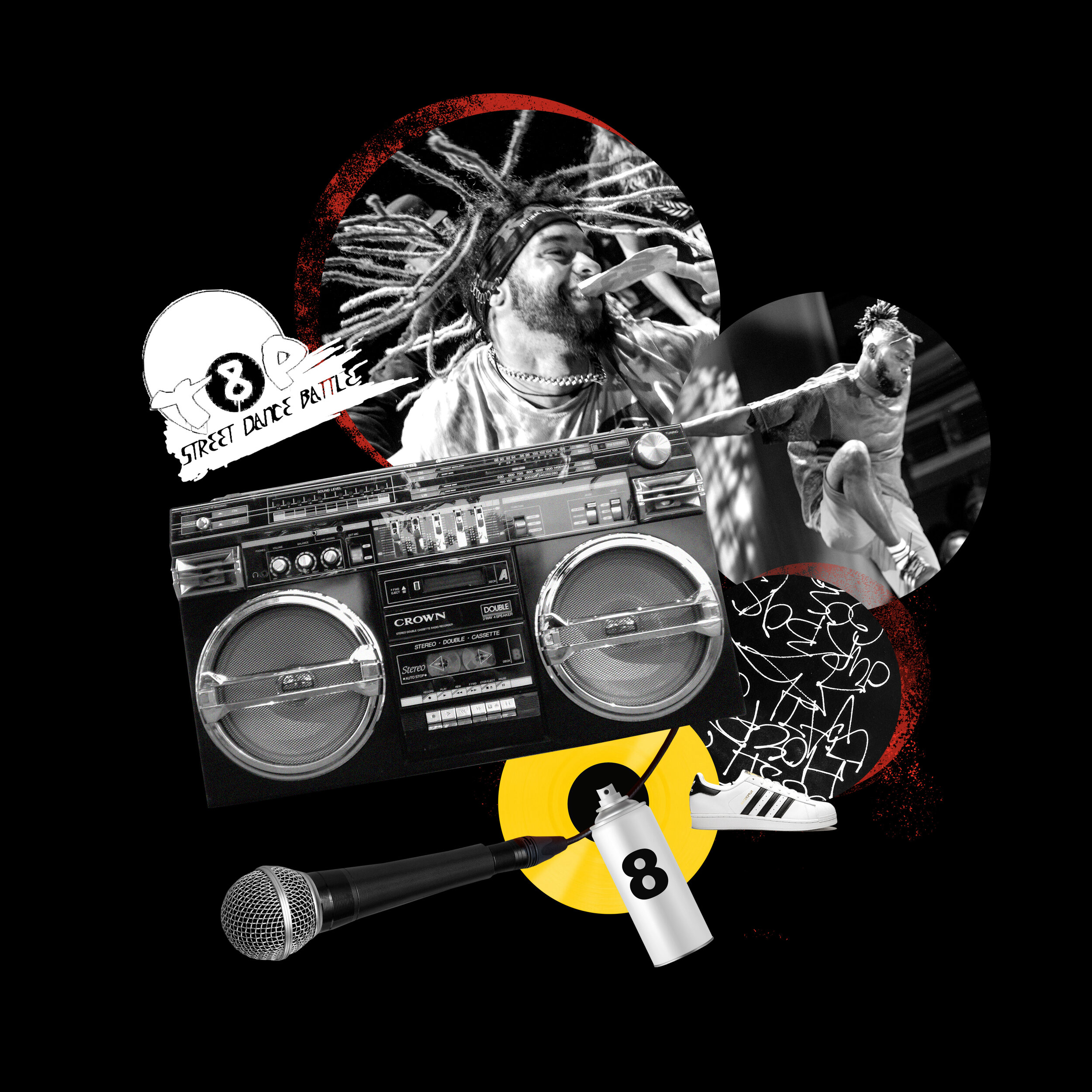This is a vibrant, collage-style poster for an urban dance battle event, set against a completely black background. Central to the image is a photorealistic black-and-white boombox labeled "Crown Dolby" on its tape deck. Flanking the boombox are various elements synonymous with hip-hop culture: a photorealistic microphone, a can of spray paint marked with the number "8", and a pair of white Adidas sneakers with black stripes and a black heel.

The poster prominently features a man pictured twice within circular frames over a subtle sliver of red. The first circle showcases him in a contemplative pose, with flowing dreadlocks and a beard, wearing a white t-shirt and a chain necklace. In the second circle, he is dynamically captured mid-jump, with one knee raised and an arm flung back, giving a sense of motion and intensity. A headband is visible, holding back his dreadlocks, emphasizing his energetic dance move.

Text elements include "T&P Street Dance Battle" written in bold, white graffiti-style letters positioned on top of the boombox. Another circle contains intricate graffiti patterns, adding to the urban aesthetic. This evocative composition, filled with imagery and symbols of street culture, conveys a fresh, energetic vibe, fitting for an exciting dance battle event.